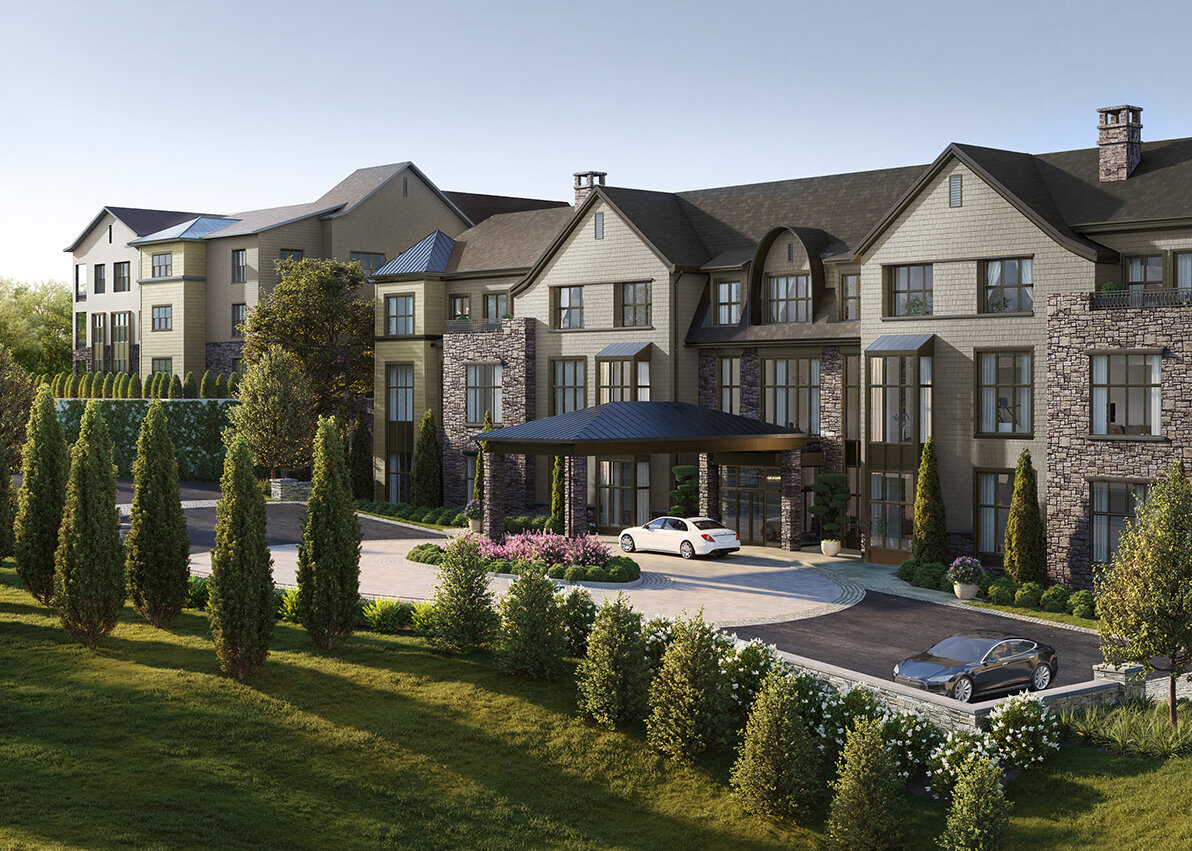This image captures the exterior of an expansive, palatial residence or possibly a high-end resort. The main building, composed of a blend of tan aluminum siding and stone elements, exhibits a modern interpretation of Tudor architectural style. The imposing structure stands three stories high and features a dark brown shingled roof adorned with multiple dormers and two brick chimneys. Tall, vertical windows with black casings punctuate the facade, adding to its grandeur.

A central carport, upheld by elegant pillars, serves as a focal point, with a white sedan parked underneath it. Flanking the carport are two gabled dormers with stone frontages, creating a balanced and harmonious visual appeal. To the left of the carport, another substantial section of the building or perhaps an entirely separate, yet similarly styled structure, extends the overall footprint of the property.

In front of the building lies a meticulously landscaped area with manicured lawns, shaped shrubbery, topiary trees, and potted flowers boasting vibrant purple blooms. The daytime setting is underscored by a bright blue sky and visible sunlight, enhancing the vivid colors and textures of the scene. The driveway, laid with asphalt, hosts a sleek black car parked to the side. Overall, the image exudes luxury and meticulous attention to detail, from the manicured greenery to the distinguished architectural elements.